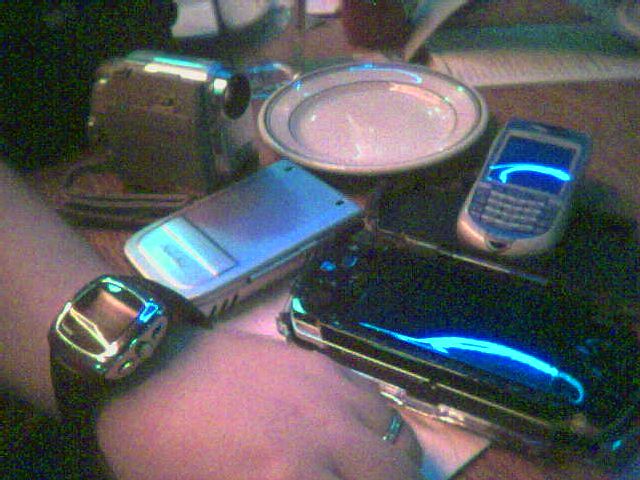In this dimly lit, pixelated photograph, we see a collection of vintage technology and miscellaneous items spread across what appears to be a diner or restaurant table. Dominating the top-left corner is a reflective, silver old camcorder, possibly an 8mm camera. To its right, there is a white plate adorned with a green stripe, next to a clear empty glass. Further right, we find a piece of paper, likely a menu, lying on the table. Below these items, an old cell phone, reminiscent of a BlackBerry, stands out with its silver buttons and a blue-silver body. Adjacent to it is another reflective item that hints at a blue light, whose exact nature is unclear. Left of this, in front of the camcorder, is another silver electronic device. The focal point, however, is the hand and wrist of a person, presumably a man, wearing a wedding band on the ring finger and a bulky, chrome watch with a black band. The watch's face is not visible due to the poor lighting. The entire scene is portrayed in a grainy, color-distorted manner that adds an air of nostalgia to the assortment of retro gadgets.